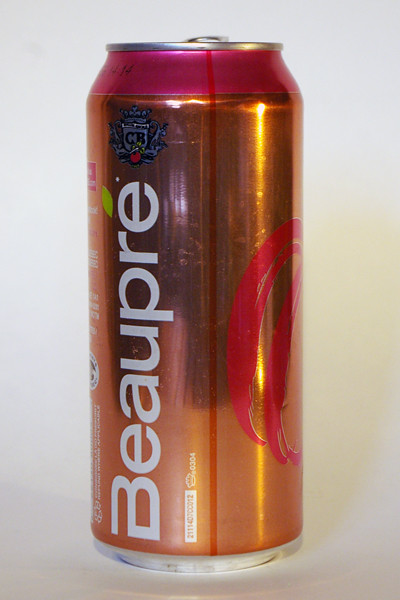The image depicts a tall, shiny, coppery-colored aluminum can with a distinctive design. The can features a wide, red brushstroke-like band encircling the top and a red circle or painted shape towards the right side. Prominently displayed on the left side of the can is the brand name "Beaupree" (B-E-A-U-P-R-E), written in bold white letters, with a small green leaf serving as an accent mark on the final "E". Above the brand name is a heraldic crest rendered in black, white, red, and gray, which appears to show a shield with the letters "C" and "R" and flanked by unicorn-like figures. The overall design gives the can a striking, chrome-red appearance, suggesting it might contain a fruit-flavored or possibly alcoholic beverage. The reflective quality of the can indicates it was photographed in an indoor setting.